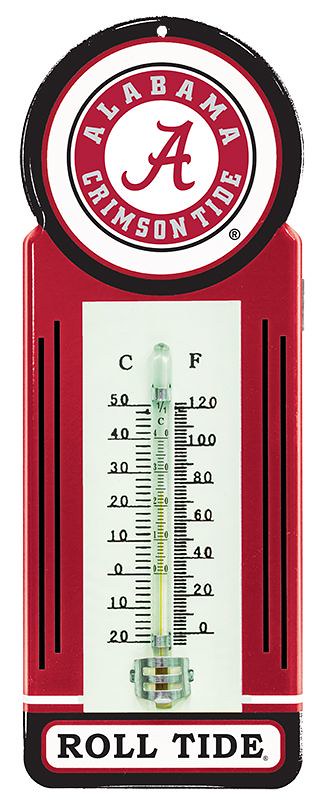This image features an ornate thermometer with a distinctive and detailed design. The thermometer is backed by a striking red background and crowned with a circular element that resembles a watch or clock face. This circular top is bordered first by a thin black line, followed by a more pronounced red line, which transitions into a larger white line, then another black line, and finally a smaller white line before reaching another red line towards its center.

In the center circle, there is white text that reads "Alabama Crimson Tide," and within this ring is a ball-shaped white circle that holds a prominent, flowing red cursive "A." The letter "A" features small feet at the bottom and has an elegant, extended crossbar that stretches both up on the left and down on the right, befitting the Alabama Crimson Tide's signature style.

Below this intricate top section, the thermometer itself is set against the red background, flanked by two thin black lines on each side. The thermometer's measurement area features a white box in the center with black numerical markings for both Celsius and Fahrenheit scales, ranging from 20 to 50 degrees Celsius and 0 to 120 degrees Fahrenheit. The temperature indicator, encased in a slightly green glass tube, stands out with a yellow line displaying the current temperature.

At the bottom of the thermometer, a black box contains a white box with red lining, and within it, the phrase "Roll Tide" is emblazoned in black letters, completing the design with a nod to the school spirit of the University of Alabama.